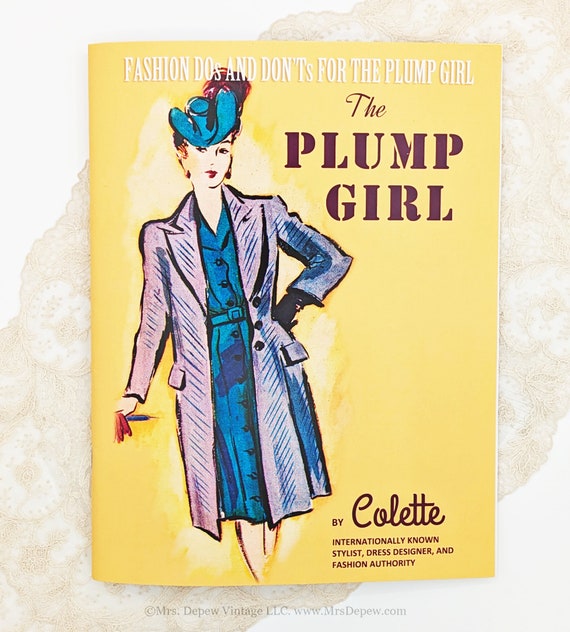The image is a color photograph depicting the cover of a vintage-styled book or magazine. The background is a white, marbled pattern with a copyright notice at the bottom reading "Copyright Mrs. Depew Vintage LLC www.mrsdepew.com". The cover has a pale yellow backdrop and features the title at the top in bold, white capital letters: "FASHION DO'S AND DON'TS FOR THE PLUMP GIRL". Just below this, in the upper right corner, is the subtitle in maroon text, "The Plump Girl". At the bottom of the cover, black text credits the author: "by Colette, internationally known stylist, dress designer, and fashion authority". To the left, an illustration of a fashionable woman commands attention. She has fair skin and is adorned in a light purple trench coat over a blue dress that fastens with buttons and has a matching blue belt around her waist. Completing her vintage look, she dons a blue hat, curved up at both sides with a red feather protruding from the back. The woman is posed with her left hand on her hip and her right hand holding a cigarette, exuding an air of elegance and timeless style.